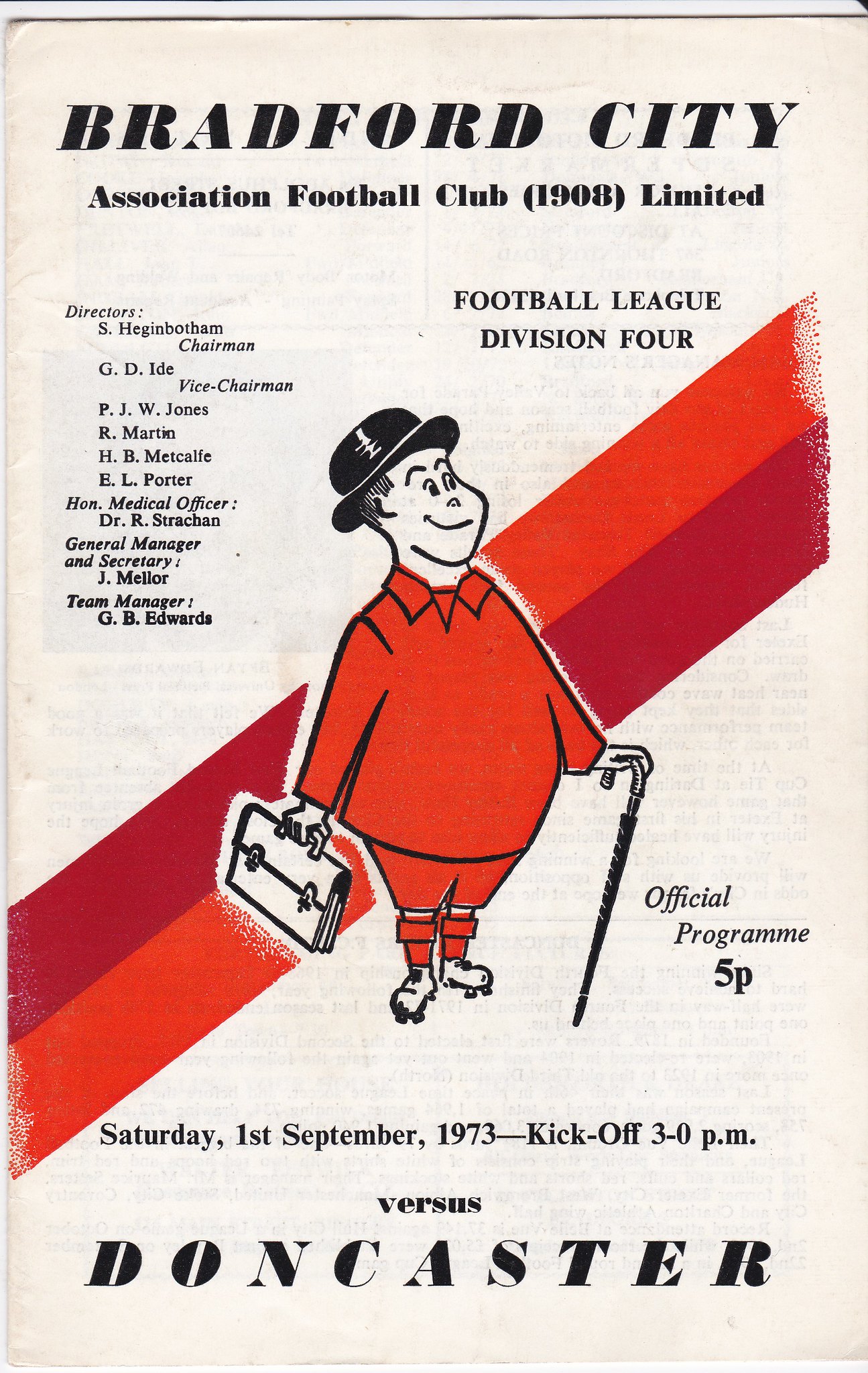The image is a vintage, black-and-white printed cover for an official football program, featuring spot color in red. At the top, bold black letters spell out "Bradford City Association Football Club (1908) Limited" followed by "Football League Division IV." To the left is a detailed list of club officers and management roles. Centered on the cover is a playful, cartoonish illustration of a rotund man with a black top hat, red shirt, red shorts, red socks, and white shoes. He is smiling and holding a white briefcase in his right hand and a black umbrella in his left, which he uses like a cane. A dark to light red diagonal stripe band runs from the bottom left to the top right, behind the illustration. Below this, "Official Program 5p" is printed, and at the bottom in bold black letters, it reads "Saturday, 1st September 1973, kickoff 3 p.m., versus Doncaster." The style echoes a classic, old-fashioned print publication.